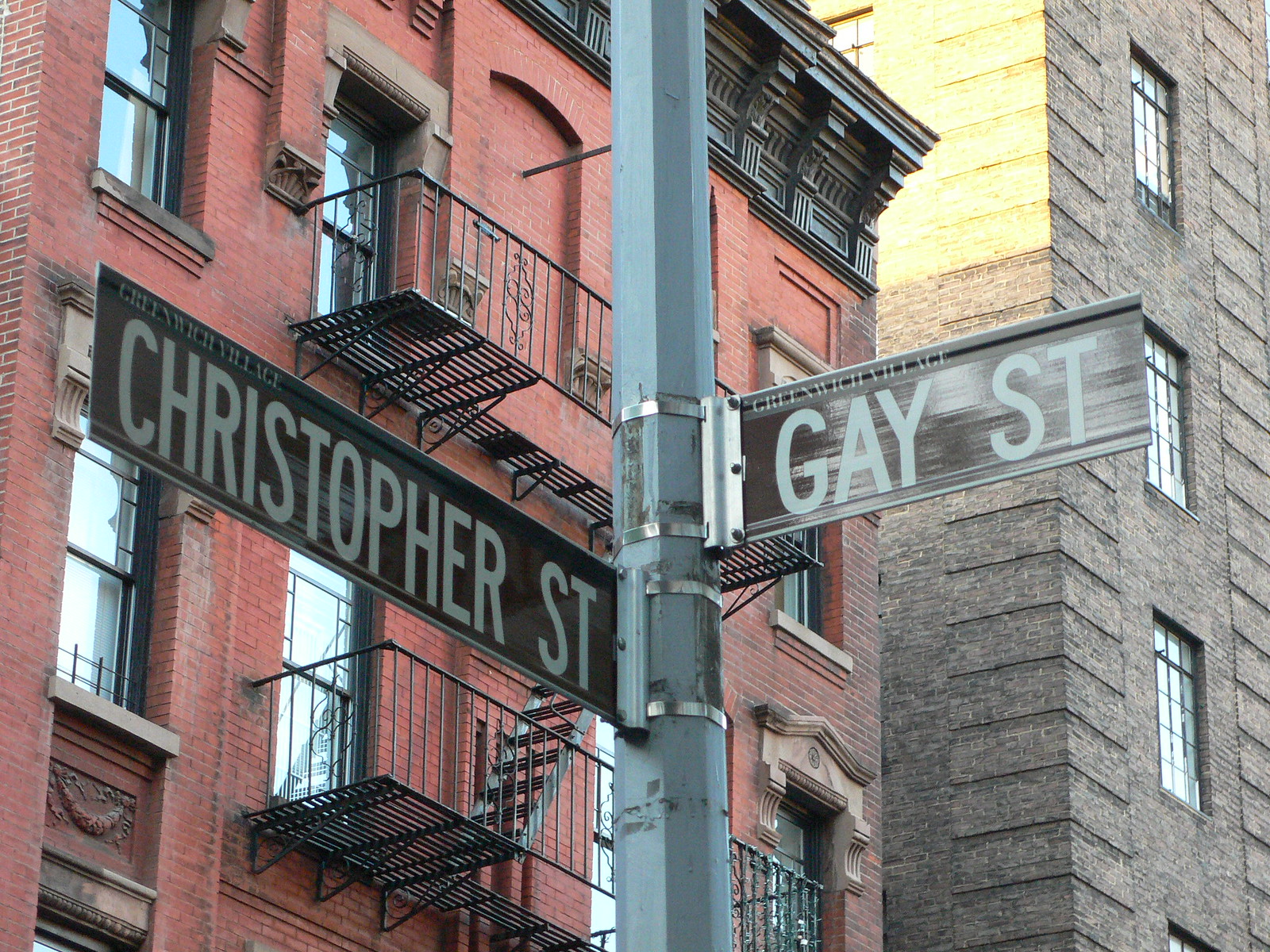This is a vibrant photograph capturing the iconic intersection of Christopher Street and Gay Street in Greenwich Village, New York City. Dominating the background is a striking red brick apartment building adorned with an array of classic black wrought-iron fire escapes. To the right stands another historic building, complementing the quintessential urban landscape. The scene beautifully encapsulates the charm and character of this famed and culturally rich neighborhood.